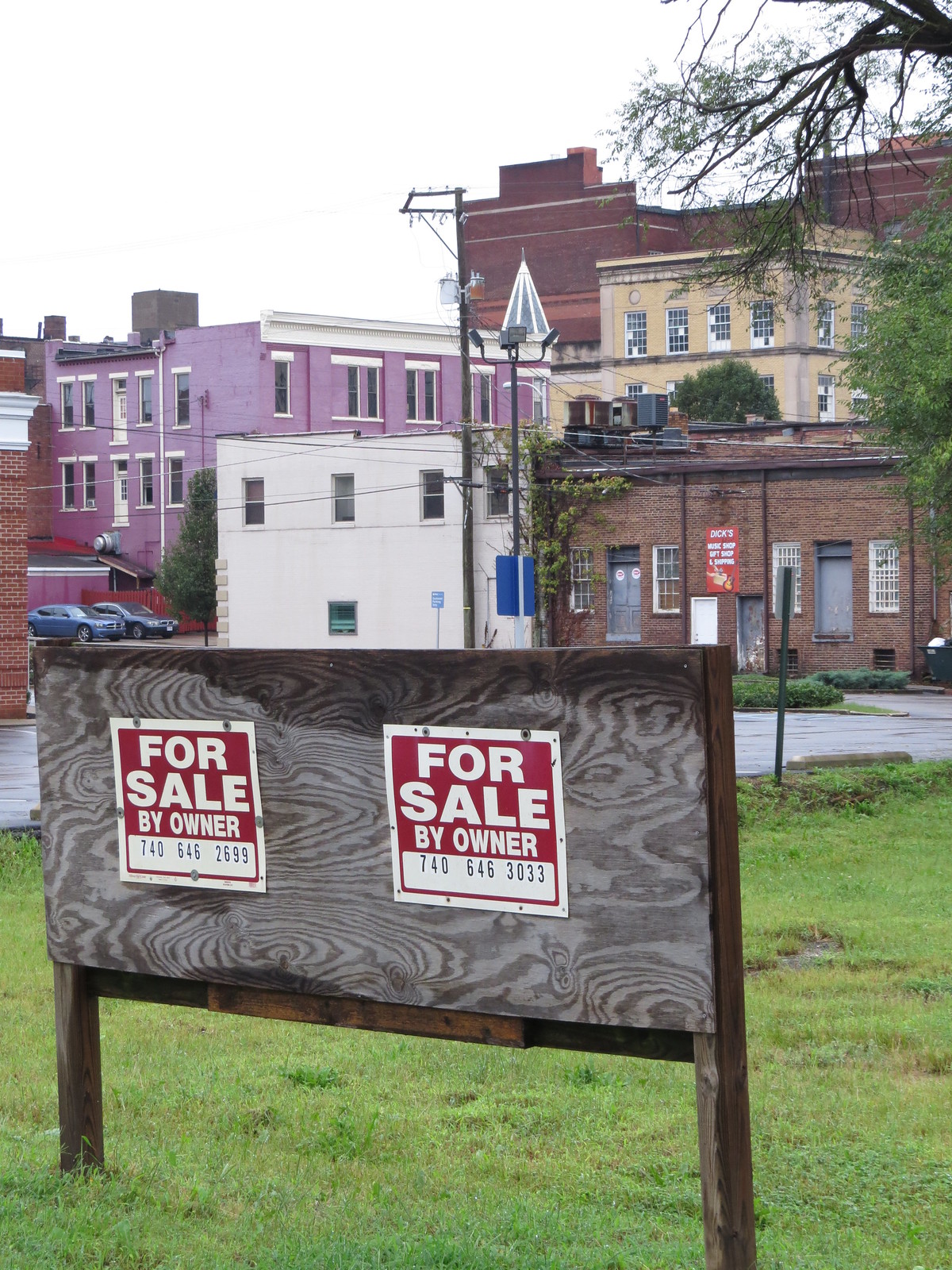The photograph captures an outdoor scene in an urban, slightly rundown shopping area. Dominating the foreground is a large grassy patch with a rudimentary sign structure made of wooden posts and a plywood base. Affixed to the plywood are two identical white-bordered signs, each showcasing a bold red square and featuring the text "FOR SALE BY OWNER" in white—one phone number reads 740-646-3033 and another mistakenly states 740-646-2699. 

In the background, a narrow street runs parallel to the grassy area, leading to a small parking lot dotted with a few vehicles, notably near a purple building. The backdrop consists of an array of worn buildings in muted colors: brown, beige, white, and purple. A partially visible sign on one building reads, “Dick’s Music Shop, Gift Shop and Shipping.” The skyline above these buildings is dreary and gray, adding to the somber mood of the photograph.

Additional elements include various traffic signs interspersed around the scene and an overarching sense of neglect hinted at by the faded facades. Despite the urban setting, the area is devoid of people, emphasizing an eerie quiet.